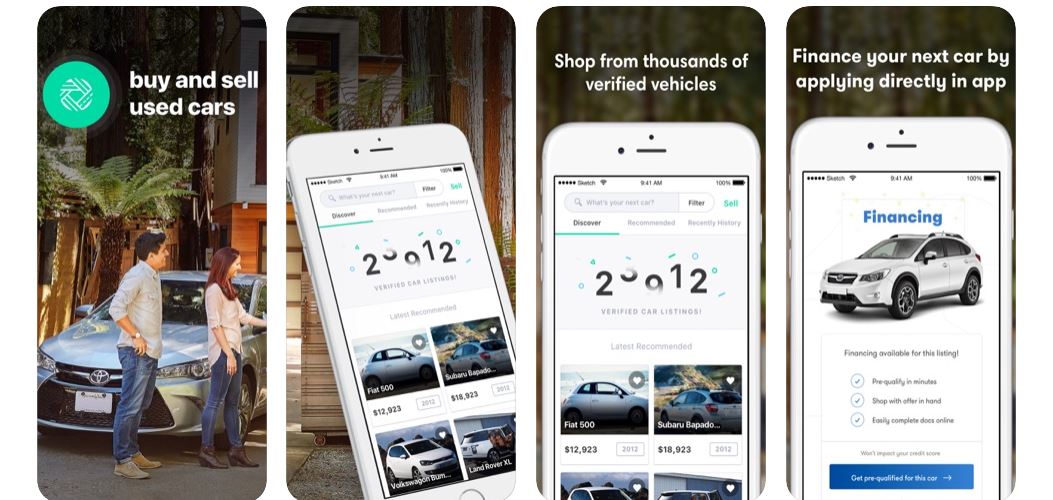This set of four images is designed to resemble cell phone screenshots and advertises a car-buying app. 

**First Image:** The background features a man and a woman, both smiling and facing towards the right, standing in front of a Toyota vehicle. A palm tree and a building are visible in the background. The top of the image prominently displays “Buy and sell used cars.”

**Second Image:** A white smartphone is shown, tilted to reveal several photographs of vehicles available for sale. Below the images, a partially cut-off number is visible along with the text “Verified car listings.”

**Third Image:** The top of the image reads “Shop from thousands of verified vehicles” and displays the same smartphone image as the previous screenshot.

**Fourth Image:** The text at the top says “Finance your next car by applying directly in app” and shows another smartphone image. The screen highlights a white four-door vehicle with the text “Financing available for this listing. Pre-qualify in minutes. Shop with offer in hand. Easily complete docs online. Won’t impact your credit score. Get pre-qualified for this car.”